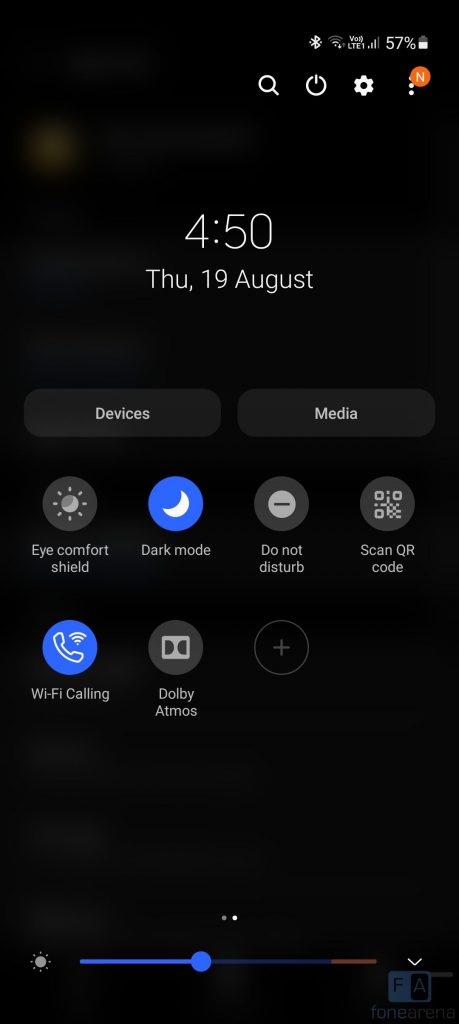This screenshot captures an Android device interface with a predominantly dark black background. In the top right corner, icons indicate that Bluetooth is active, Wi-Fi connectivity has 2 out of 4 bars, cellular signal is on LTE with 3 out of 4 bars, and the battery level is at 57%. Just below these icons are additional controls including a magnifying glass (likely for search), a power button, settings, and notifications.

The time is displayed prominently at 4:50 on Thursday, 19th of August. Directly beneath the time, gray buttons labeled "Devices" and "Media" are positioned side by side.

Further down, a series of shortcut icons are presented for quick access to various features. These include Eye Comfort Shield, Dark Mode (highlighted in blue, indicating it is active), Do Not Disturb, Scan QR Code, Wi-Fi Calling (also highlighted in blue), and Dolby Atmos. A faint plus sign encased in a circle is situated next to Dolby Atmos, suggesting the option to add another app to the main screen.

At the bottom of the screen, the brightness control slider is visible, set to approximately 42%, with a drop-down button positioned to its right.